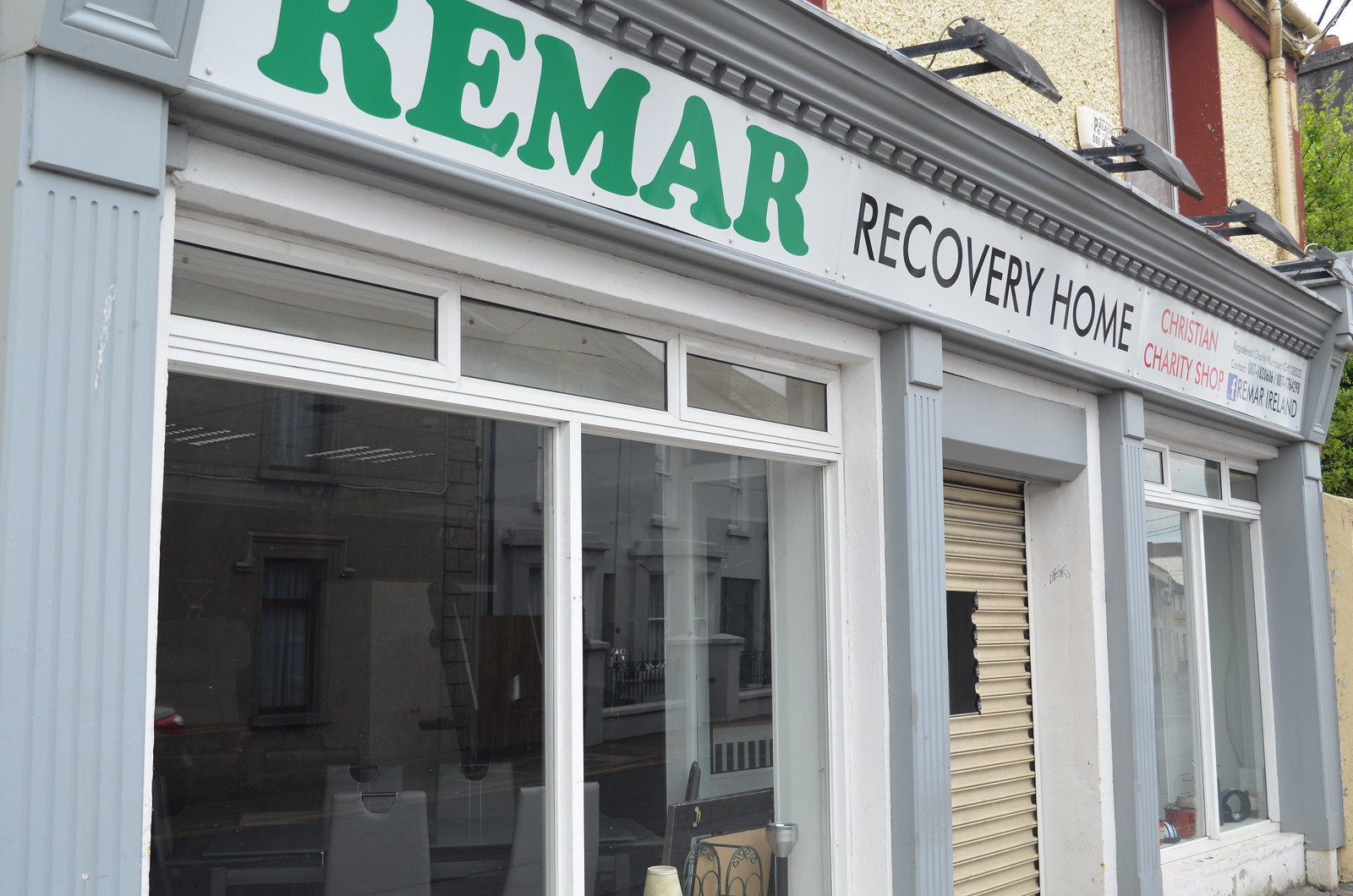The image depicts the closed entrance of an old, gray and white storefront in what appears to be a European country. The building features four large, white-framed windows and a solid, shuttered front door situated between two of these windows. Above the door, a white banner displays the store's information in a sequential manner: "Remar" in green text, "Recovery Home" in black text, "Christian Charity Shop" in red letters, and the phrase "Registered Charity Number" in black letters, which is partially illegible. Additionally, the banner includes a Facebook logo followed by the text "Remar Island." Mounted on the roof, downward-pointing exterior lights illuminate the sign. The store, seemingly out of business, stands as a testament to its former role as a charitable organization within the community.